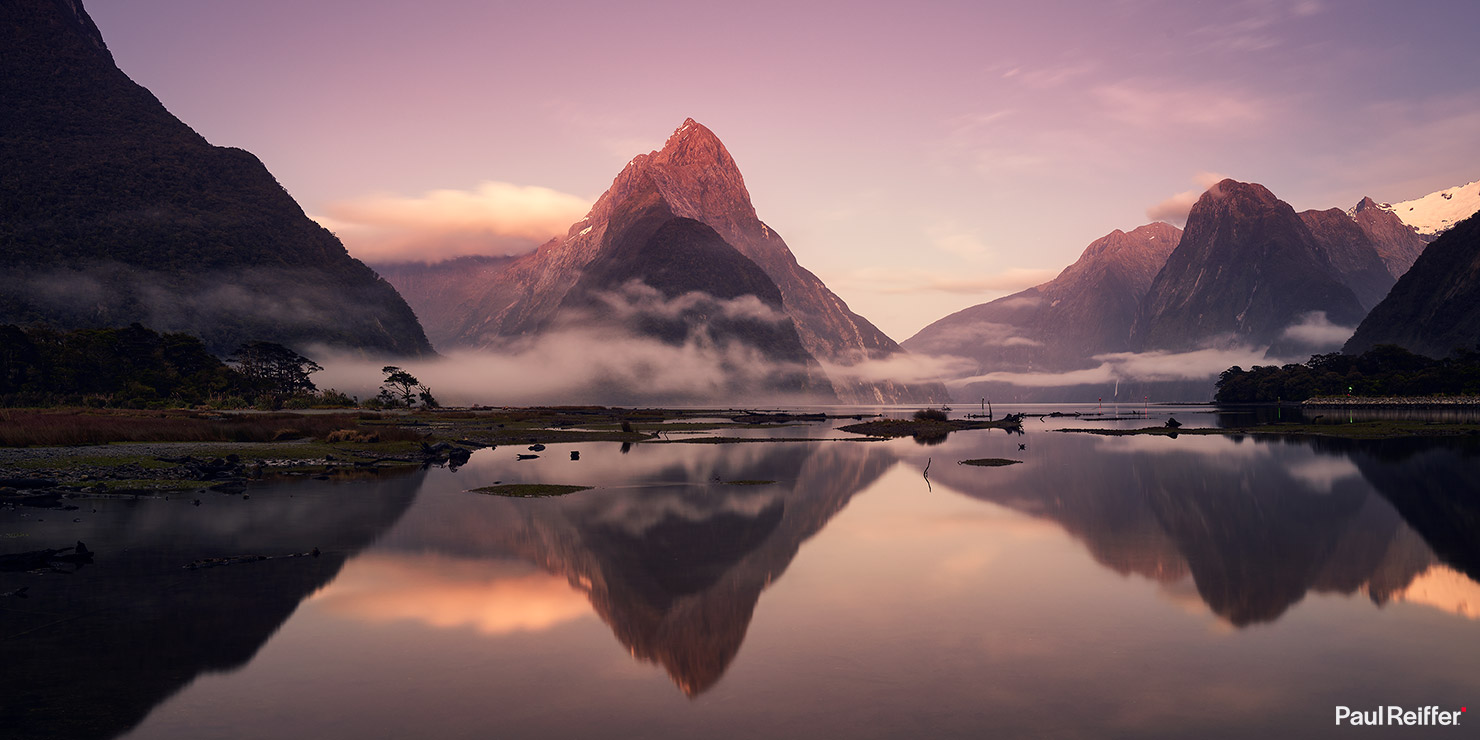In this captivating photograph by Paul Reifer, a striking landscape unfolds at either dawn or sunset, highlighted by a rich purple and pink hue permeating the sky. The scene features a serene lake with crystal-clear, dark waters that mirror the vivid backdrop of majestic mountains. These mountains exhibit a blend of bright brown and purple shades, with billowing clouds cascading towards the ground, enhancing the dreamlike quality of the image. To the far left, distinctive trees—reminiscent of those found in Africa, with slender trunks and sparse, tufted foliage—add an exotic touch. The lake itself is dotted with small, sandbar-like islands, enriching the complexity of the vista. The photographer's signature, "Paul Reifer," is elegantly inscribed in white, sans-serif font in the bottom right corner, grounding this ethereal scene in a professional presentation.